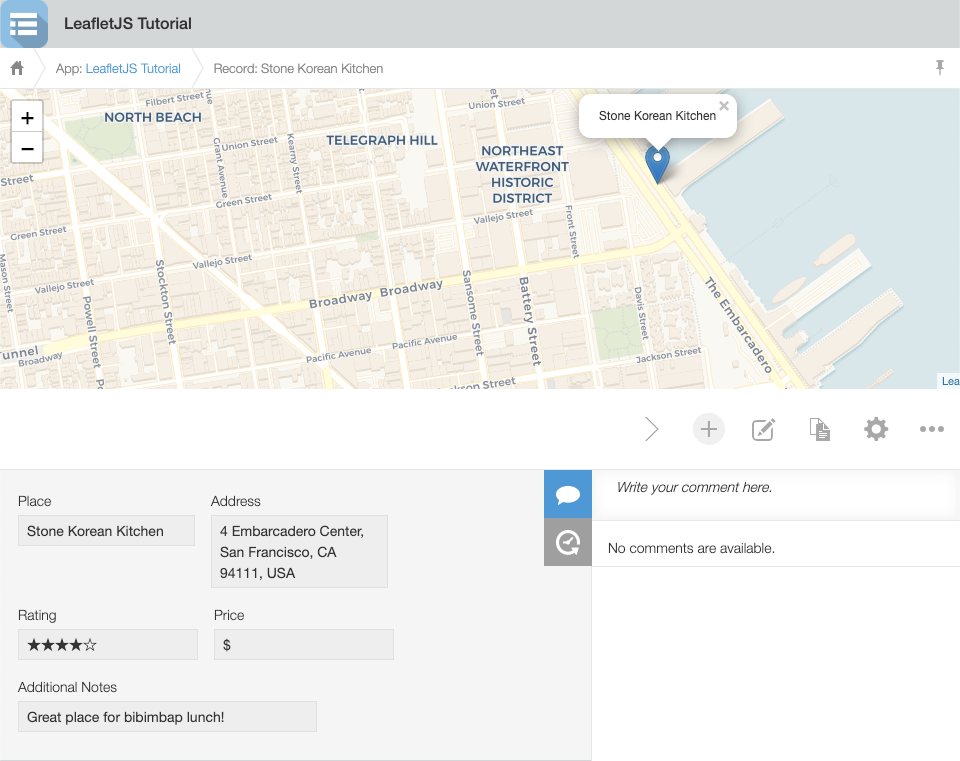A detailed screenshot displaying a map interface, primarily tinted in blue with white lines marking routes. Positioned in the upper left corner are three horizontal lines, with two of them featuring adjacent dots. Adjacent to these lines on the right, there's a text header that reads "Leaflet JS Tutorial." Below this header, the main map occupies the majority of the screen, presenting an aerial view.

On the left side of the map, there's a vertical toolbar including a plus-minus icon for zooming in and out, and a house icon above it for returning to the homepage. A title bar just below this toolbar reads "App Leaflet JS Tutorial" in blue. The map itself is clearly detailed, showcasing road names and specific locations. Notably, "Stone Korean Kitchen" is marked, and the "Northeast Waterfront Historic District" appears in capital letters in one section. Other notable locations include "Telegraph Hill" and "North Beach," both in capital letters. Toward the right side of the map, there's a label that begins with "Embargo" and continues with partially obscured text.

On the right side of the interface, there's a side menu containing an arrow icon, a pencil icon, paper icons, a settings icon, and a three-dot menu. Just below, there's a search bar where the term "Stone Korean Kitchen" is entered along with an adjacent address. Next to this, there's a chat bubble and an arrow icon with the prompt "Write your comment here," indicating no available comments. Below these elements is a rating section displaying four out of five stars, a single dollar sign as the price indicator, and a section labeled "Additional Notes" containing the text "Great place for bibimbap lunch."